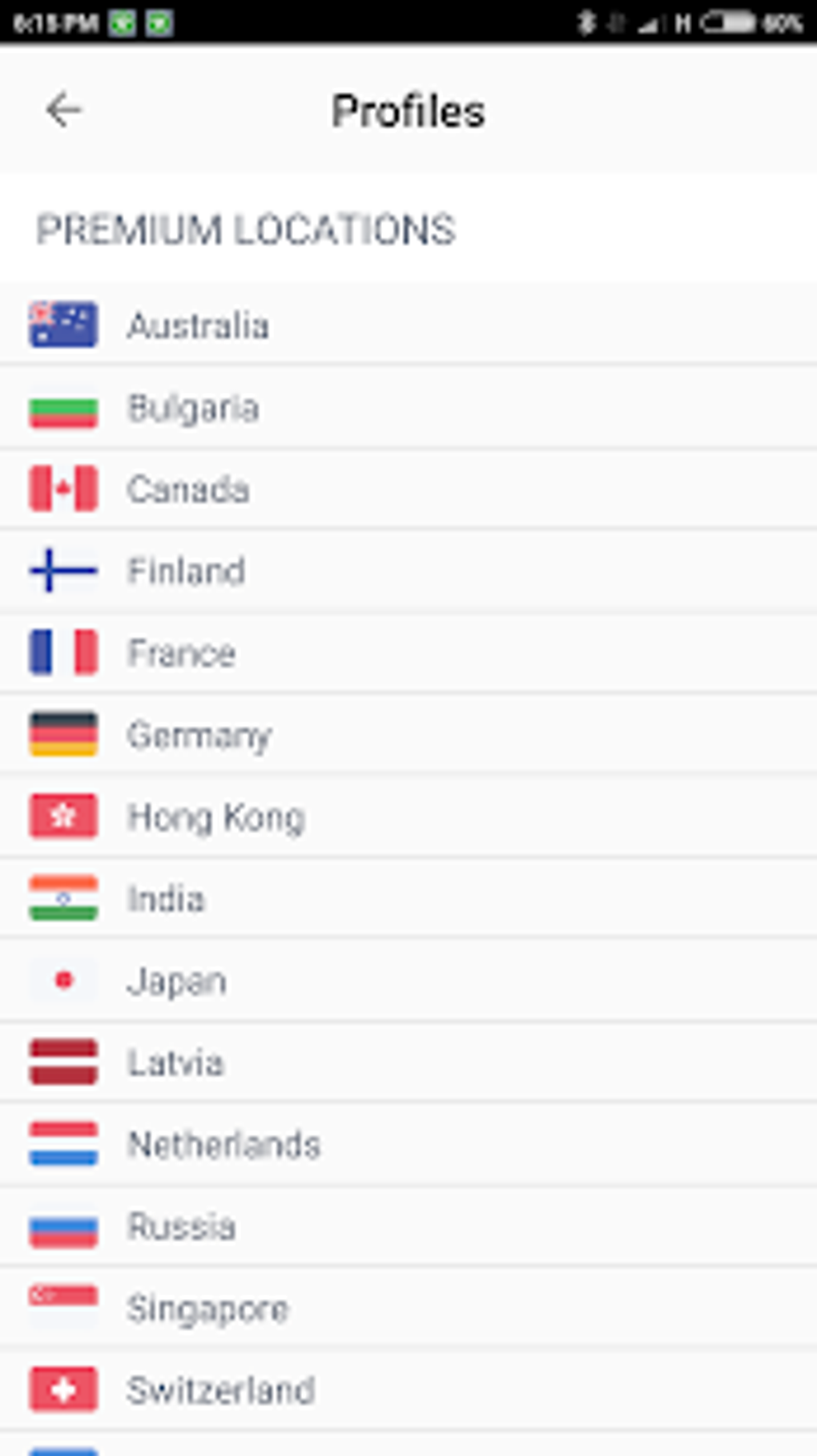A blurry screenshot of a mobile phone screen, captured at 6:15 p.m., displays an interface with two indeterminate green icons at the top. The battery icon shows a 50% charge, with normal network bars and Bluetooth icons also visible. Below these, the screen reads "Profiles," indicating a list of selections followed by a back button. The main content showcases "Premium Locations," listing countries alongside their respective flags. The nations displayed include Australia, Bulgaria, Canada, Finland, France, Germany, Hong Kong, India, Japan, Latvia, Netherlands, Russia, Singapore, and Switzerland, with an additional partially visible flag at the bottom hinting at another country. The countries are organized in individual gray bars separated by thin lines, resembling piano keys against a white background.